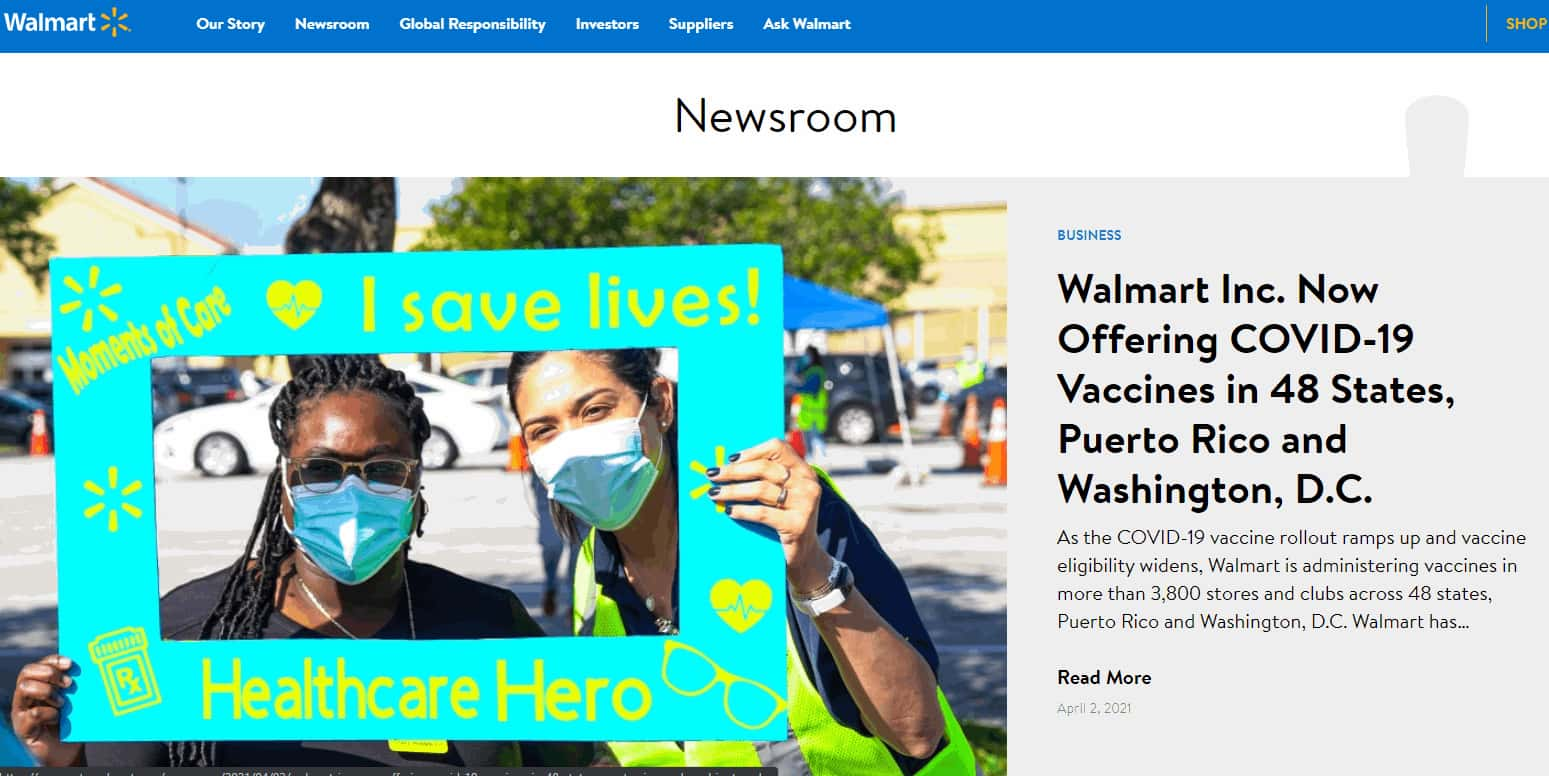Screenshot of Walmart Website Newsroom Page

In this detailed screenshot captured from the Walmart website, the top left corner features the recognizable Walmart logo, accompanied by its signature yellow star. A prominent blue navigation banner stretches across the top, containing tabs labeled: Our Story, Newsroom, Global Responsibility, Investors, Suppliers, and Ask Walmart.

The title of the webpage is clearly marked "Newsroom" in bold black text at the top. Below this title, a large, engaging photo occupies a significant portion of the screen. The image showcases two Black women, both wearing blue protective face masks commonly used during the COVID-19 pandemic. They are joyfully holding up a neon blue poster with a rectangular cutout in the middle; their heads peek through the opening. The poster is adorned with vibrant yellow text that reads: "Moments of Care, I Save Lives, Healthcare Hero," surrounded by charming graphics like glasses, heartbeats, and EKG lines, along with the Walmart logo.

To the right of the image, under the category title "Business," the main article is introduced with the headline: "Walmart Inc. now offering COVID-19 vaccines in 48 states, Puerto Rico, and Washington DC." The accompanying description reads, "As the COVID-19 vaccine rollout ramps up and vaccine eligibility widens, Walmart is administering vaccines in more than 3,800 stores and clubs across 48 states, Puerto Rico, and Washington DC. Walmart has..." followed by an ellipsis, indicating more content. Just below this text, a "Read More" link invites further exploration, and the date "April 2, 2021" is noted in smaller text beneath it.